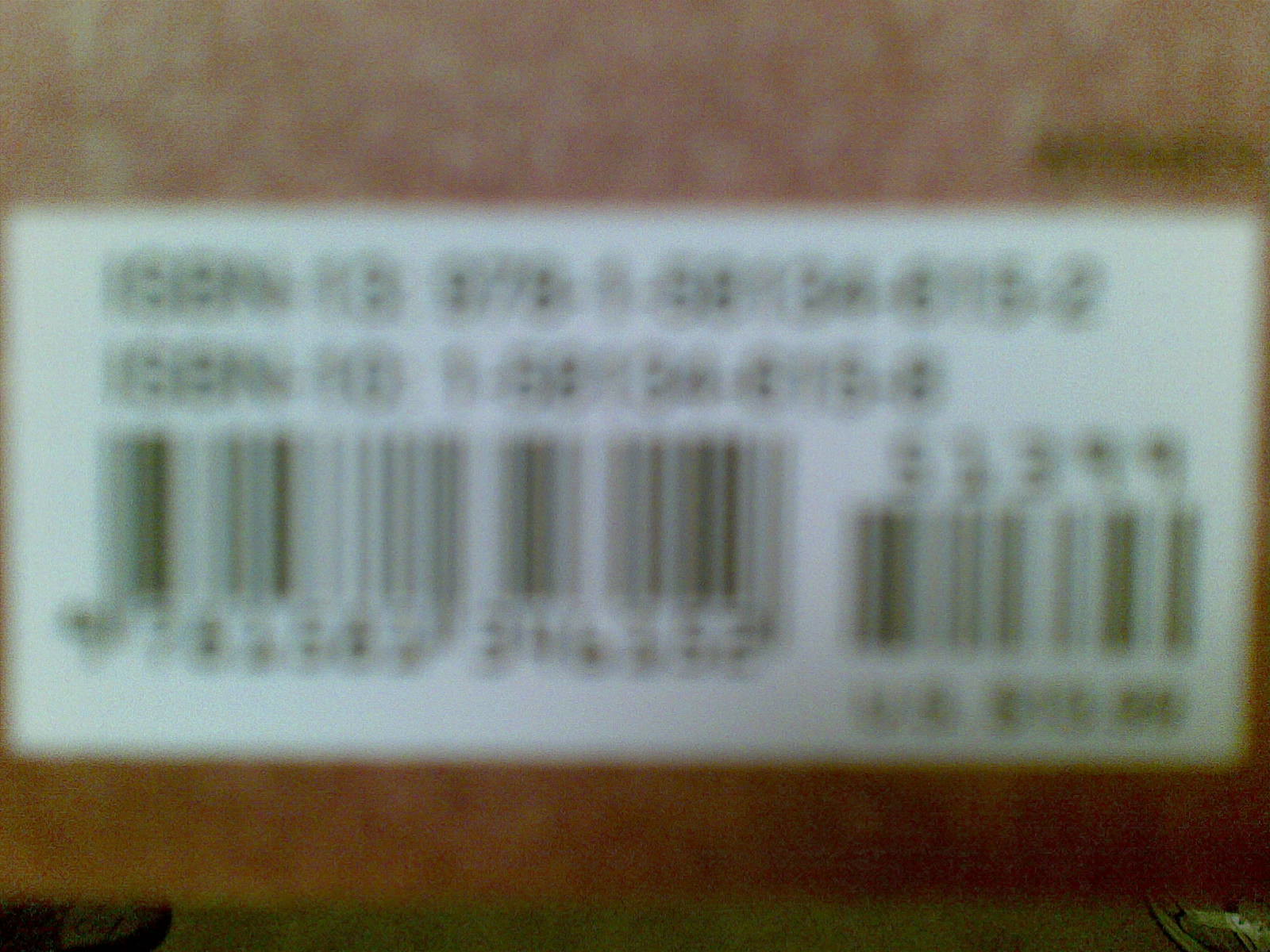The image depicts a very blurry and out-of-focus photograph of a white rectangular sticker set against a background that transitions from a reddish-orange or gold shade to a brown color at the bottom. At the top of this sticker, there are two rows of serial numbers, which are not legible due to the poor quality of the photo. Below these rows are two barcodes, each accompanied by a series of numbers beneath them. The barcode on the right has an additional set of numbers above it. The background appears pixelated, creating an impression of a building exterior, although it's not definitively clear due to the extreme blurriness and close-up nature of the shot. The image also shows something green in the top right corner, though its identity remains undetermined. Overall, the photograph focuses on the white label with barcodes and numbers, all rendered unreadable by the image's poor resolution.